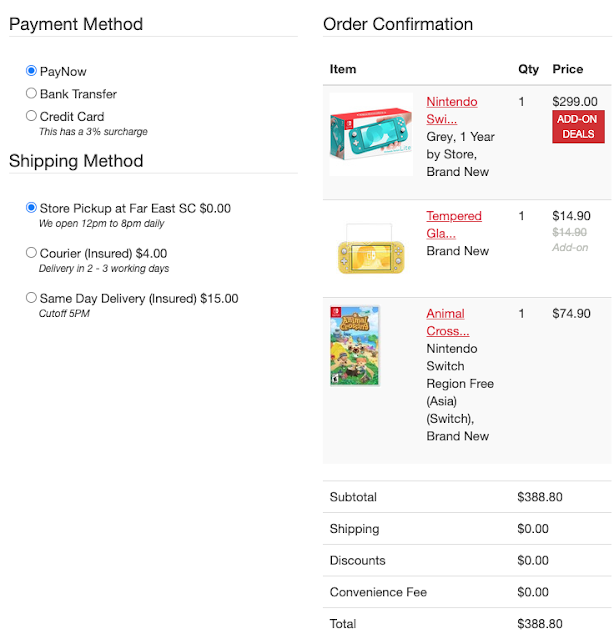**Detailed Caption for Website Checkout Page Image:**

The image is a screenshot depicting a website's detailed checkout page. On the left side of the screen, there is a vertical column outlining the payment and shipping information. The first section is titled "Payment Method," which includes three clickable buttons: "Pay Now," "Bank Transfer," and "Credit Card." Notably, the "Credit Card" option mentions a 3% surcharge. The "Pay Now" button is currently selected. Below this section, there is another titled "Shipping Method," which offers three choices: "Store Pickup at Far East SC" (costing $0 and available daily from 12 p.m. to 8 p.m.), "Courier Insured" (costing $4 with a delivery timeframe of 2 to 3 working days), and "Same Day Delivery Insured" (costing $15 with a cut-off time of 5 p.m.). "Store Pickup at Far East SC" is the selected option.

On the right side, there is an "Order and Order Confirmation" section. This area lists three columns labeled "Item," "Quantity," and "Price," detailing the purchased products. 

1. **First Item:** 
   - **Image:** A box featuring a handheld gaming device.
   - **Description:** Nintendo SWI (presumably Switch), Grey, 1 Year, by Store, Brand New.
   - **Quantity:** 1
   - **Price:** $299

   There is also a red box beneath this item labeled "Add-on Deals."

2. **Second Item:**
   - **Image:** Another handheld device.
   - **Description:** Tempered Glass, Brand New.
   - **Quantity:** 1
   - **Price:** $14.90
   - Additionally, a grayed-out text beneath it mentions "$14.90 Add-on."

3. **Third Item:**
   - **Image:** A game.
   - **Description:** Animal Crossing for Nintendo SWI, Region Free, Asia, Brand New.
   - **Quantity:** 1
   - **Price:** $74.90

Below the item listing, details of the overall order costs are provided:
- **Subtotal:** $388.80
- **Shipping:** $0
- **Discounts:** $0
- **Convenience Fee:** $0
- **Total:** $388.80

This comprehensive breakdown gives a clear picture of the items purchased, the chosen payment and shipping methods, and the total cost of the order.